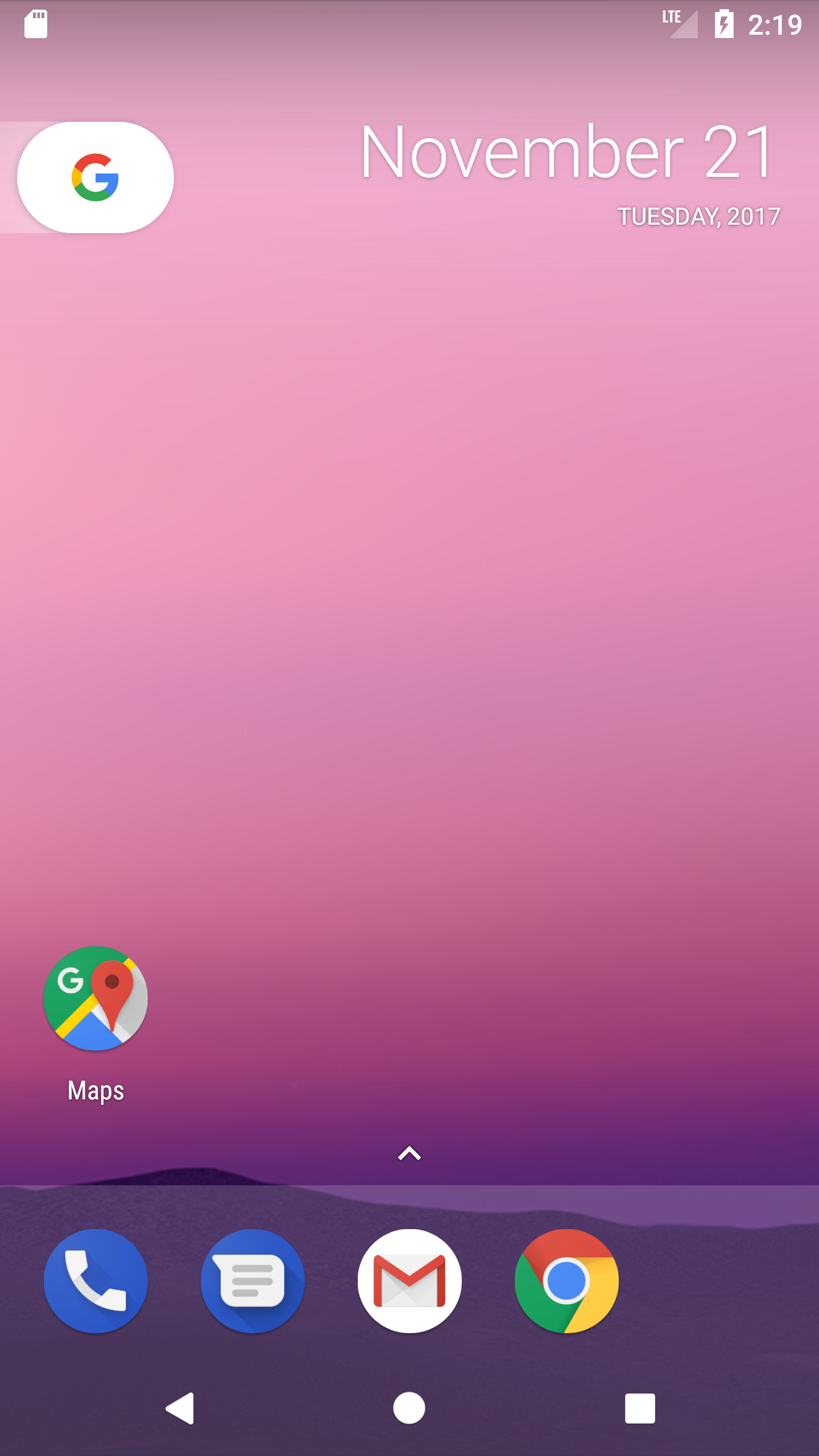The image is a screenshot of a phone screen featuring a gradient background. The top portion, extending from the top to about two inches from the bottom, displays a violet gradient that is slightly darker at the top and bottom edges, giving it a shadowy effect. The bottom two inches transition to a deep, dark purple, with a subtle streak of lighter purple coming in from the right and fading halfway across the screen.

In the top left corner, there is a small square missing its top left corner. To its right, there is text reading "2:19," next to a battery icon indicating that it is charging. The LTE symbol appears next to an empty triangle.

On the left side of the screen, there is a white Google search bar. Inside the bar, the Google 'G' logo is displayed in its signature colors: red at the top, yellow on the left, green on the bottom, and blue on the right. To the right of the 'G,' the date "November 21" is written in white text, with "Tuesday, 2017" in smaller lettering underneath.

At the bottom left of the violet gradient, there is a divided circle. A yellow line splits this circle diagonally from the top right to the bottom left. The top left section of the circle is green and features a white 'G.' Below this, there is a large red location icon, with the top half of the right side colored light blue and the bottom half dark blue. Beneath the icon, the word "apps" is written in white text.

In the center of the violet section, there is a greater-than sign (>) pointing upwards. Below this symbol, in the deeper purple area, there are four app icons lined up horizontally. The first icon is blue with a white phone symbol, the second is blue with a white message icon, the third is the Google email icon, and the fourth is the Google Chrome icon.

At the very bottom of the screen, slightly to the right of the center, there is a sequence of navigation buttons including a left-pointing triangle, a circle, and a square, all in white.